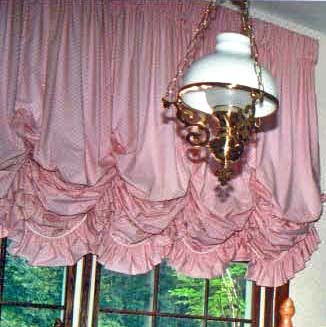This detailed image captures the interior view of a house, focusing on a close-up of a window adorned with pink, silk-like curtains cascading from the top to the mid-section of the window. These curtains feature three tiers of ruffles and are elegantly gathered in various places, creating a layered effect. The window itself is encased in brown paneling with distinct brown mullions, beyond which lush green trees are visible. Notably, there is a small, ornate chandelier suspended from the ceiling by a golden chain, featuring a circular white top and golden hardware, dangling toward the middle right-hand area of the image. The ceiling is white, while the adjacent wall is also painted white. The chandelier appears to have a singular bulb and is delicately outlined by three chains that add to its refined appearance.